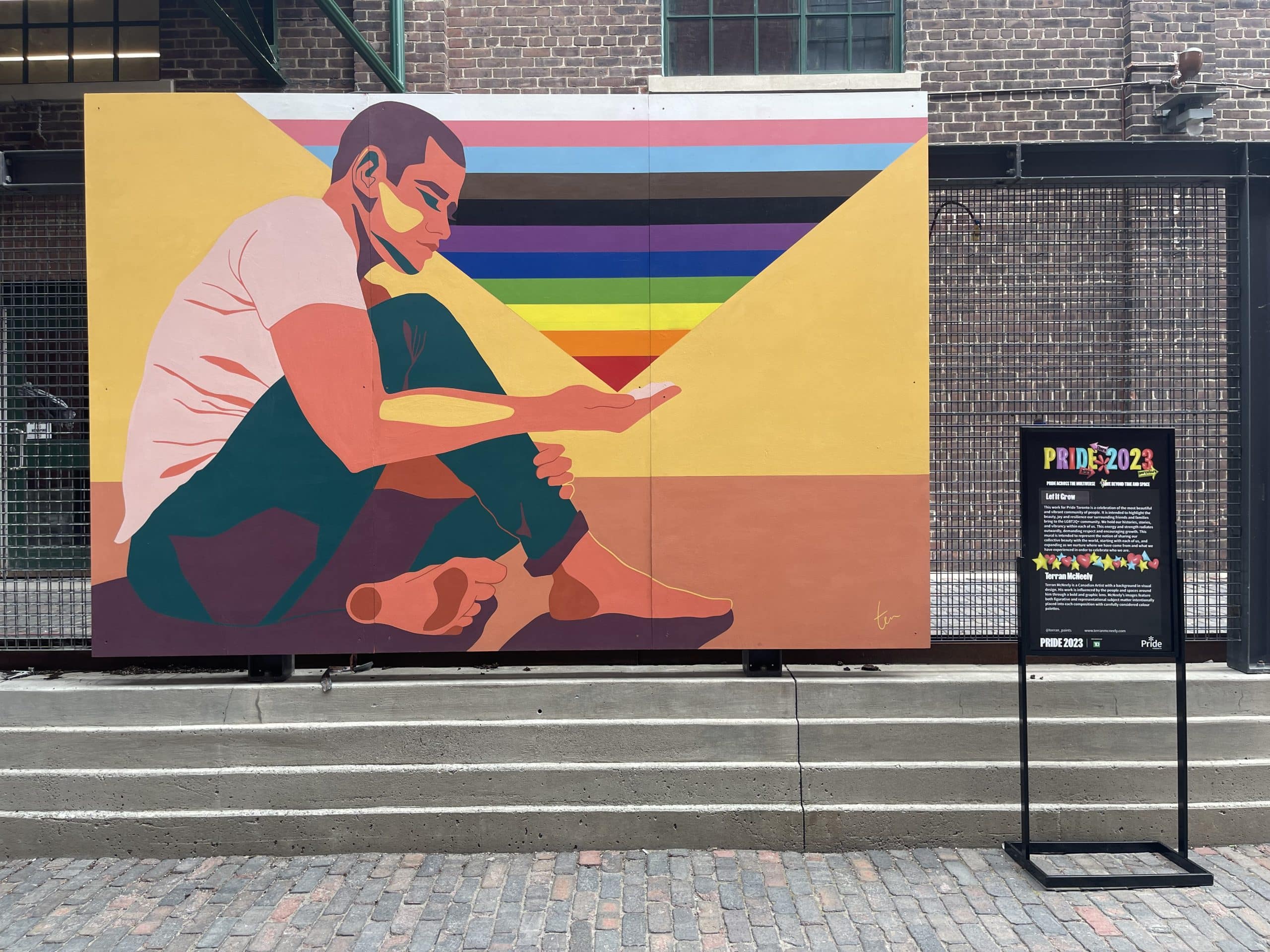The mural depicted in the image is a vibrant pride painting titled "Let It Grow" by artist Taron McNeely. Positioned on a brick wall at the top of a staircase, the painting features a young, barefoot man with a shaved head, dressed in a white shirt and blue sweatpants. He is seated and gazing contemplatively down at his right hand, from which an upside-down triangle with rainbow-colored stripes emanates. The triangle begins with red near his hand, followed by orange, yellow, green, blue, and violet, and transitions into a mix of black, gray, light blue, pink, and white at its peak. The mural is framed by a black gated fence on either side, with a small plaque to the right that reads "Pride 2023," providing further details about the piece and its creator. The mural's background includes a brick building and windows, integrating the artwork seamlessly into its urban setting.